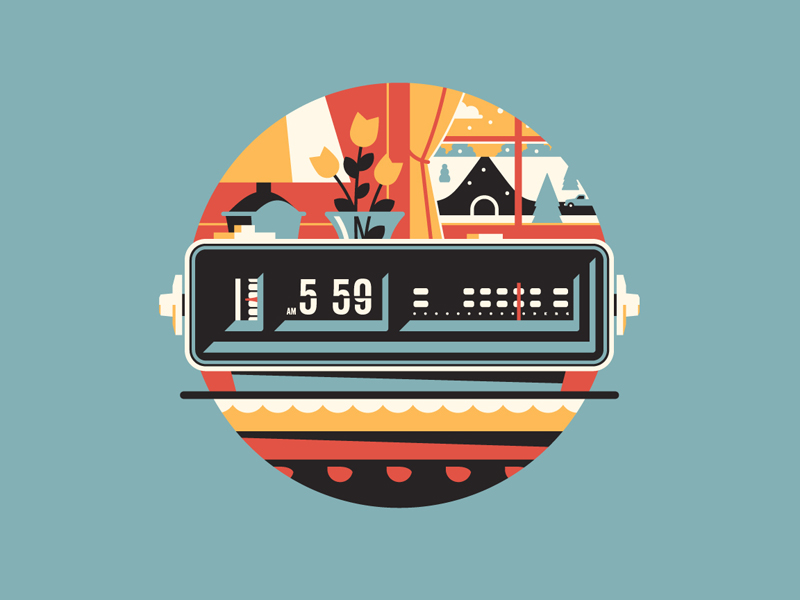This image appears to showcase the front panel of a highly decorative radio. The design is unique, featuring unconventional oblong indicators instead of traditional round dials. On the left side, the number "559" is prominently displayed. To the far left, there is a narrow slot functioning as a marker dial, which is highlighted by a vertical red line. Adjacent to the numbers, another set of graduations is marked with a similar red line. The top section of the panel features stylized imagery within a circular motif, showcasing intricate designs of flowers and possibly other natural elements.